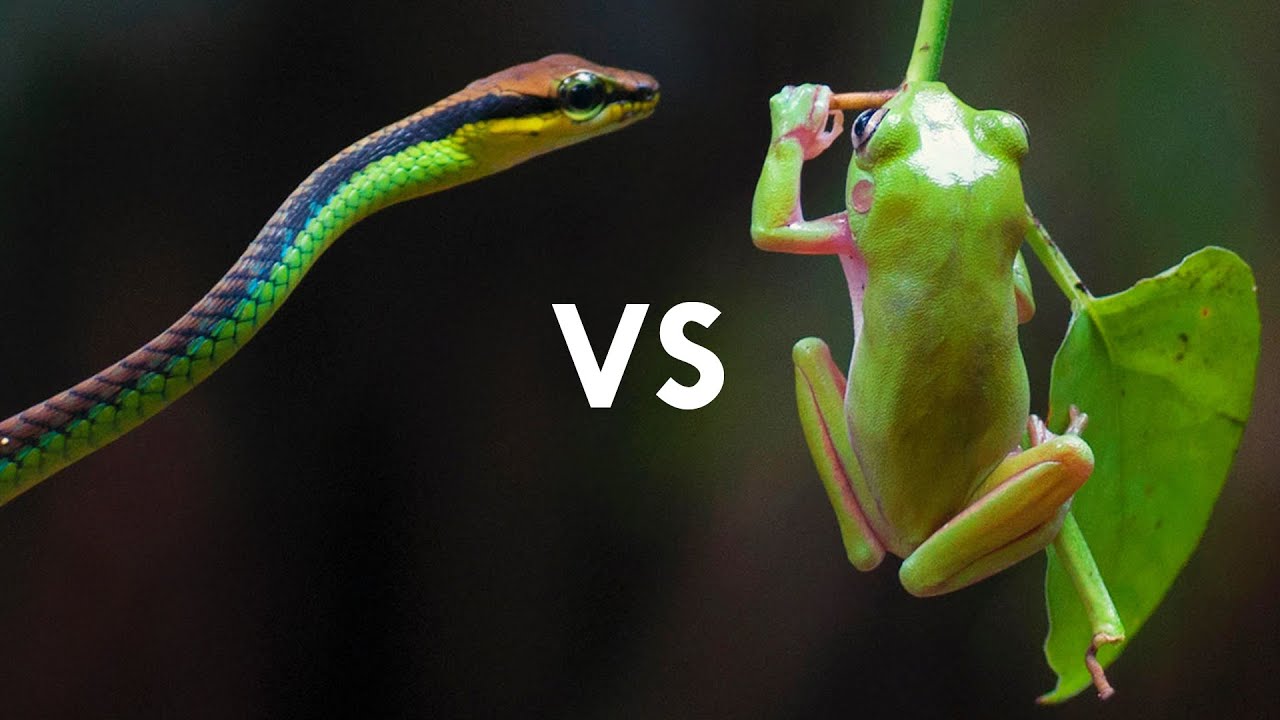This horizontal, professional nature photograph captures a vivid scene featuring two colorful creatures seemingly poised in a dramatic encounter. On the left side, a strikingly colored snake commands attention with its vibrant hues of red, blue, green, and yellow, punctuated by a large, expressive eye. Its body, thin and elongated, appears to be angled towards the right. To the right, a green tree frog, with pinkish plum accents on its underside and limbs, clings to a branch and leaf. The sharply focused subjects stand out against a blurred green background, which may be digitally manipulated to enhance their presence. Dominating the center of the image, large white text reads "VS," implying an impending showdown between the snake and the frog. While the authenticity of the interaction is questionable, the image powerfully conveys a sense of confrontation in the wild.